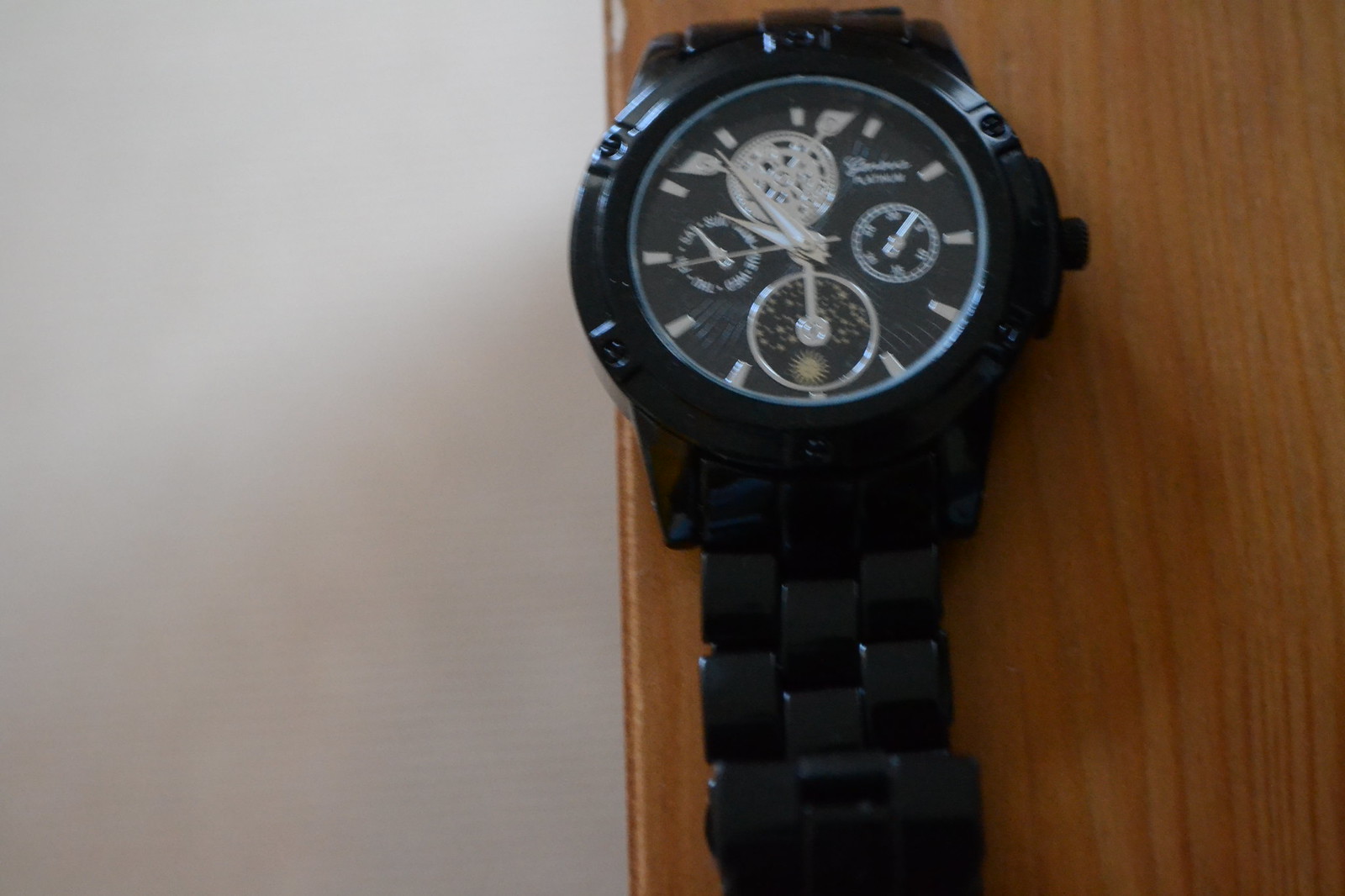The image depicts a black wristwatch with a sleek, plastic-like band, positioned at the edge of a wooden table. The background on the left side of the image features a large, off-white, almost gray wall, contrasting with the wooden surface. The watch itself has a black face, enclosed in a glass cover. Time is marked by small dashes without any numerical indicators, corresponding to five-minute intervals. There are four smaller dials set into the black face of the watch. The top dial appears to contain gears, while the dial at the three o'clock position has small numbers that don’t resemble a traditional clock. Another dial, located near where the six o'clock mark would be, contains celestial elements like stars and a sun, and the final dial near the nine o'clock position has indistinguishable numbers. The watch hands and smaller indicators are silver, contrasting against the dark background. Additionally, the watch face includes the manufacturer's name which starts with an "L" and the word "platinum." The current time displayed on the watch is approximately six minutes past ten o'clock. The watch also features a knob on its right side.